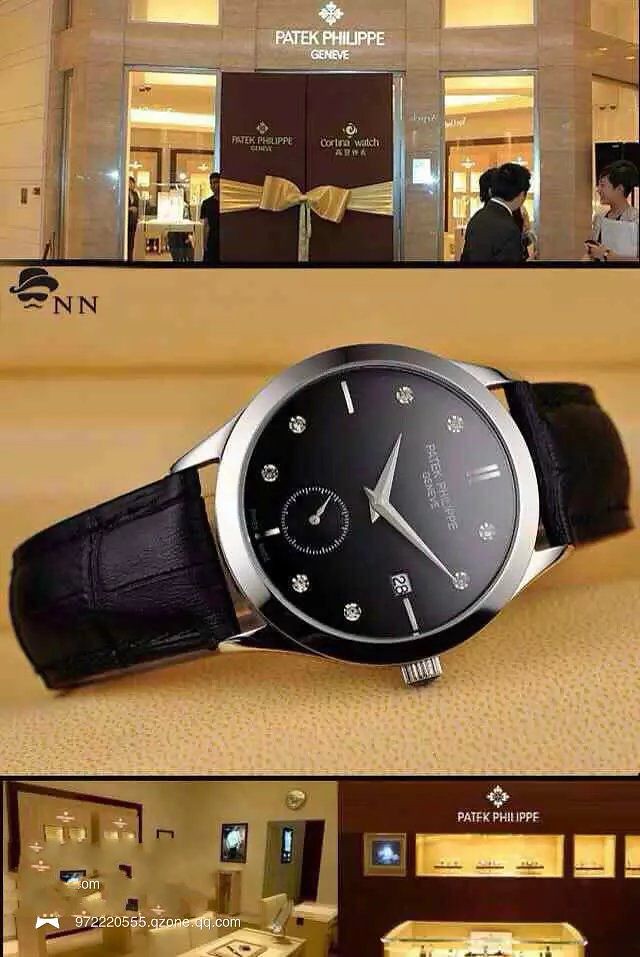In this compilation of photographs, the centerpiece is a striking close-up of a luxurious Patek Philippe wristwatch from Geneva. The watch features an elegant black face adorned with the brand's distinctive logo, encased in polished silver or stainless steel. Its sophisticated look is amplified by a black leather band, exuding classic sophistication. Adding a touch of opulence, small diamonds are meticulously placed at the 2, 4, 6, and 8 o'clock positions on the watch face. Surrounding the central image are additional photos capturing a storefront adorned with a large ribbon at the front door, suggesting a grand opening event or a special occasion, adding context and dimension to the scene.